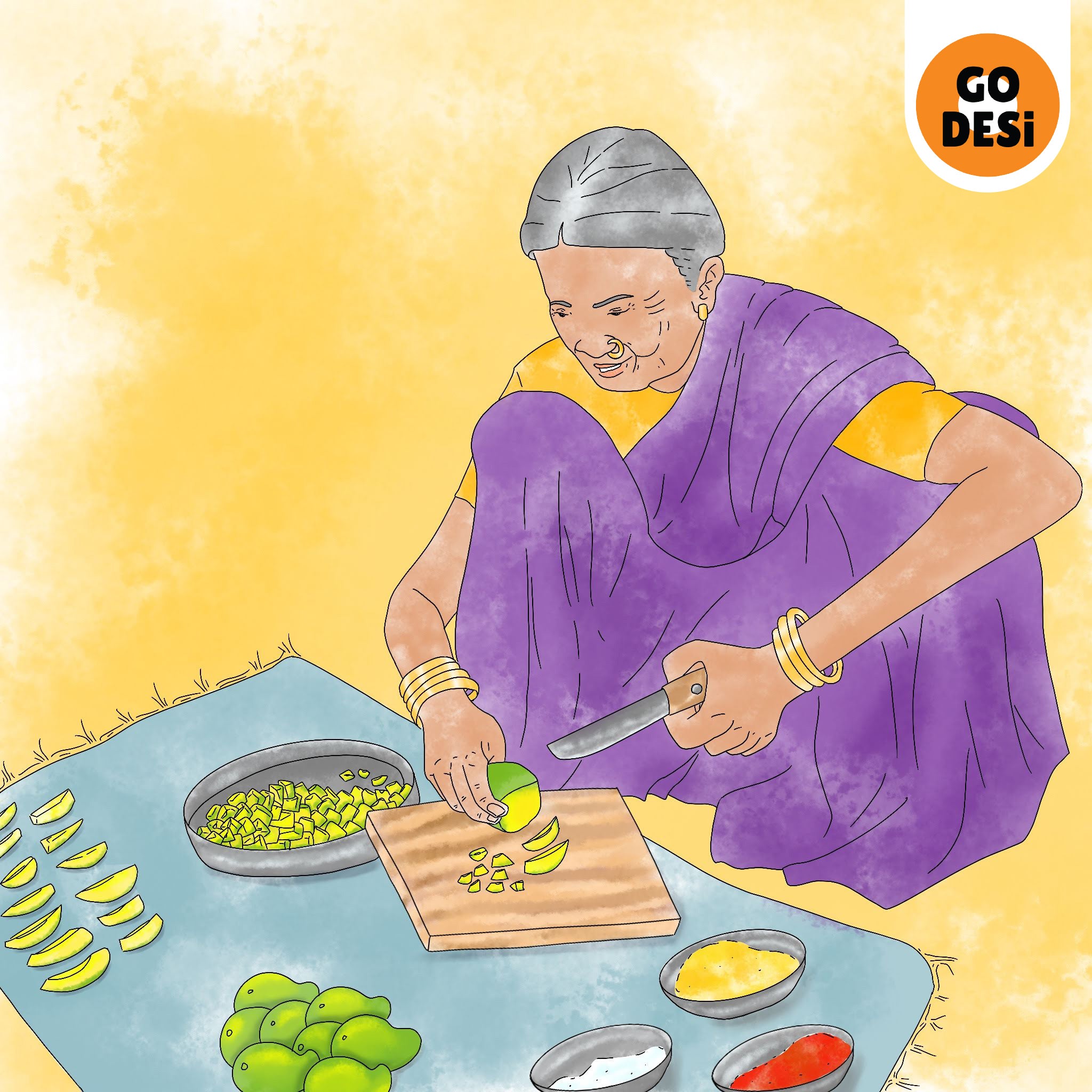This detailed illustration captures an older South Asian woman with gray hair, tied back in a bun, as she prepares a meal on the ground. She is dressed in a traditional attire with a short-sleeved yellow shirt beneath a flowing purplish robe that envelops her lower body. Her accessories include several golden bracelets—four on the right wrist and three on the left—a gold nose ring, and a gold earring in her left ear. 

Crouched over a blue cloth mat, the woman is cutting a green fruit, likely pears or mangoes, using a knife in her left hand. Chunks of this fruit are being placed into a silver tub beside her. Surrounding her on the mat are more slices of the green produce, and a wooden cutting board used for chopping.

To her left are three silver dishes filled with different spices: one yellow, one white, and one red. The background is an airy, watercolor yellow, creating a warm atmosphere. In the top right corner, an orange circle with a white center prominently displays the text "Go Desi" in black.